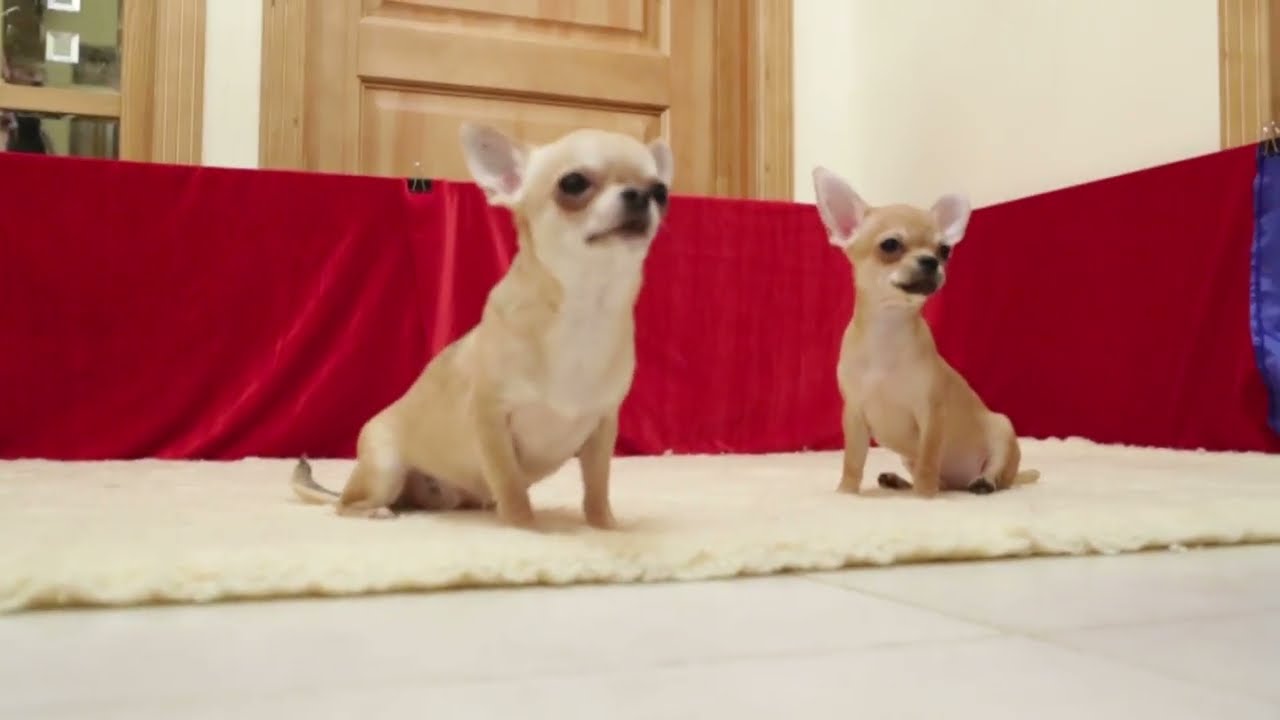This photograph captures two baby chihuahuas sitting on a small piece of cloth that separates them from a white tile floor. Both are enclosed by a makeshift barrier, a red cloth held upright by clips creating a cozy but contained area for the puppies. The chihuahua on the left has its ears perked up attentively, as if it just heard a sound, and is looking directly at the camera. The chihuahua on the right, slightly larger, has its ears somewhat erect and is gazing straight ahead, possibly at the photographer. This red-clad enclosure sits within a room featuring a wooden door and a window with a matching wood trim, suggesting the puppies are closed off in this space, making it a potential setup for an advertisement to sell the young chihuahuas.